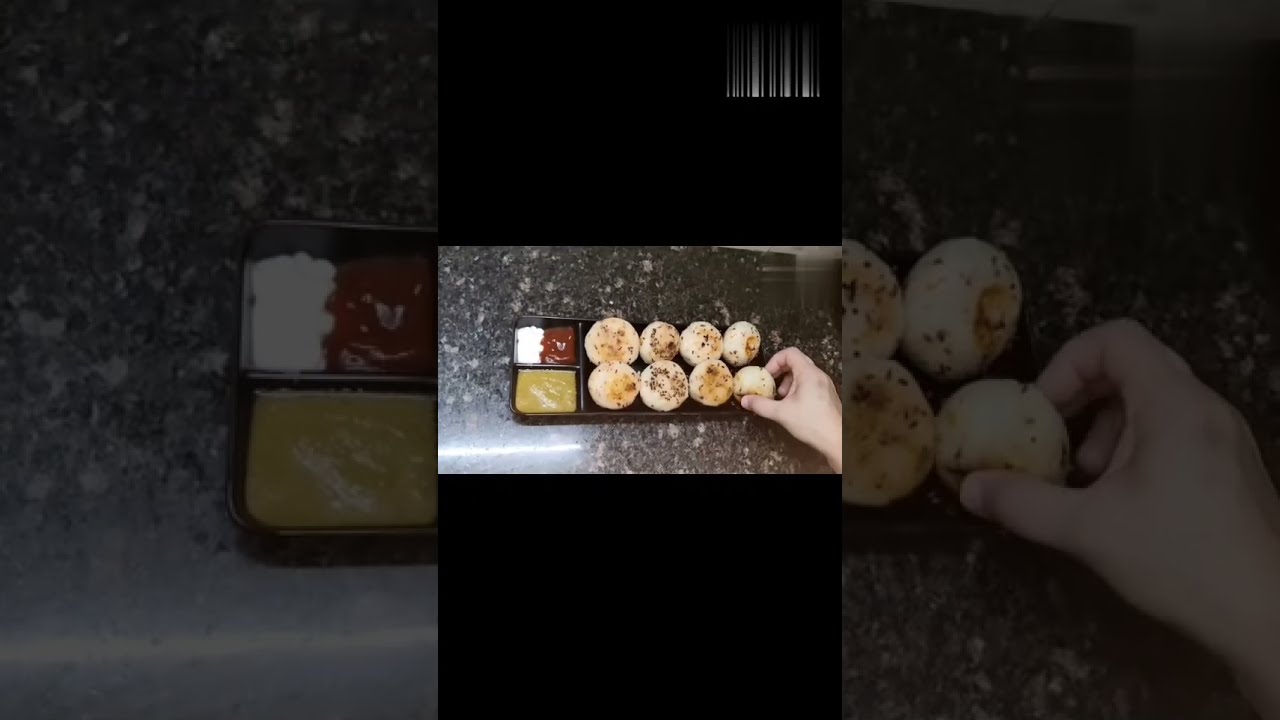The image showcases a vertically oriented, three-panel composite. The outer left and right panels are darkened and contain close-up versions of the central image, which is brighter and positioned at an angle. The central rectangular image features a dark marbled kitchen countertop with a black plastic tray containing food. The tray has multiple compartments: a longer one on the right filled with eight spherical, doughy balls, possibly dumplings or pastries with poppy seeds. A hand reaches in from the right side, grasping one of the doughy balls. To the left of this compartment are three smaller sections with condiments. The bottom compartment appears to contain mustard or honey mustard, the middle one holds what looks like ketchup, and the top has a white condiment that could be mayonnaise or rice. The entire composition is bordered by long black bars at the top and bottom.